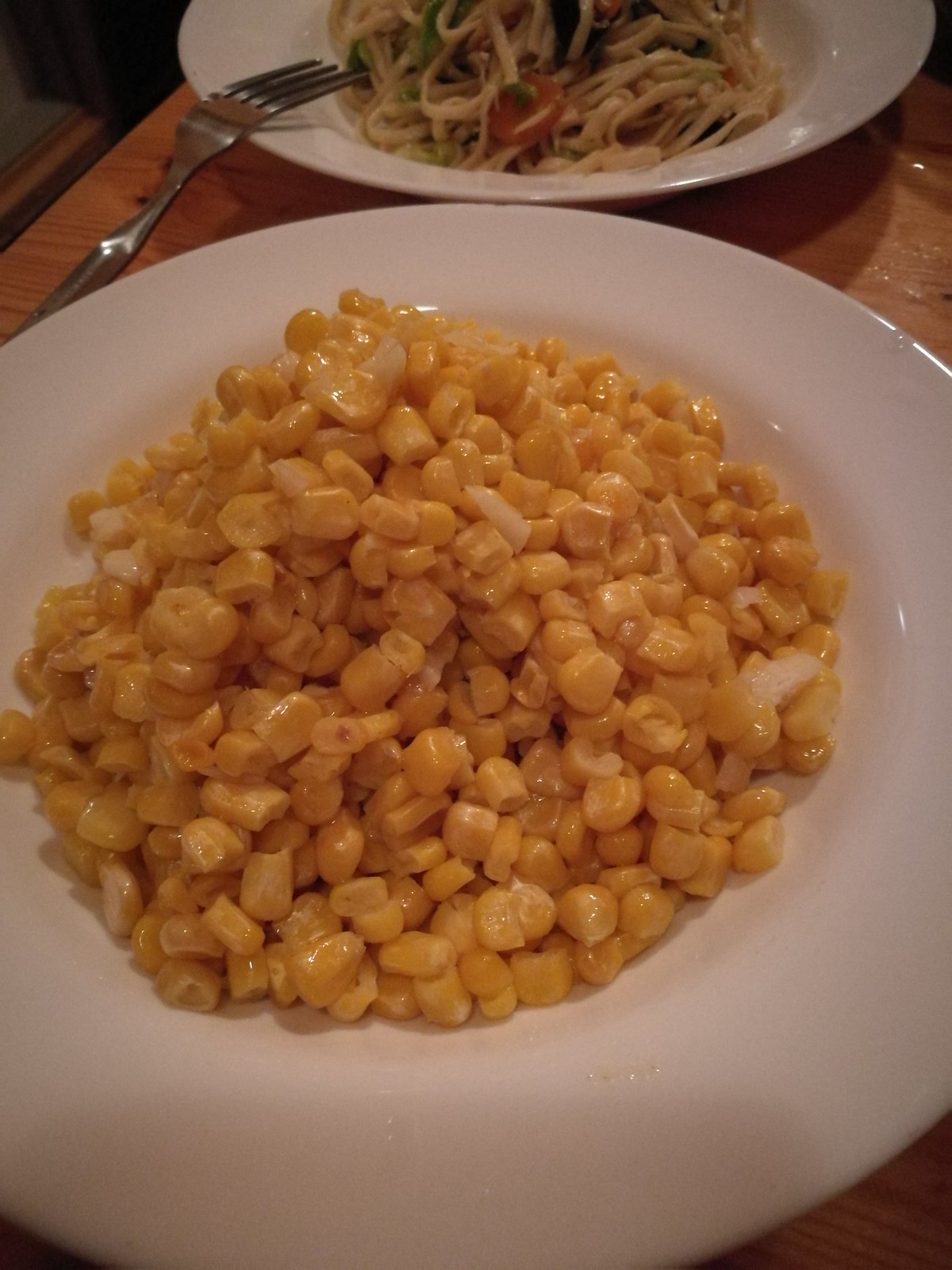In this image, we see a dining setup on a light brown, woodgrain-finished table. Dominating the foreground is a large white ceramic bowl filled with cooked sweet corn niblets, some of which have slightly browned. The corn appears to be seasoned, possibly with butter or oil. Behind this bowl, occupying the upper portion of the photograph, is another white porcelain bowl containing a pasta dish. This pasta seems to be a mix of noodles, carrots, peas, and potentially some greens, with a piece of tomato suggesting a hint of red amidst the ingredients. A fork is casually leaning against the edge of this pasta bowl. The background features part of a chair positioned against the table, indicating a relaxed dining environment, possibly either a cozy home kitchen or an indoor restaurant setting with warm yellowish lighting.